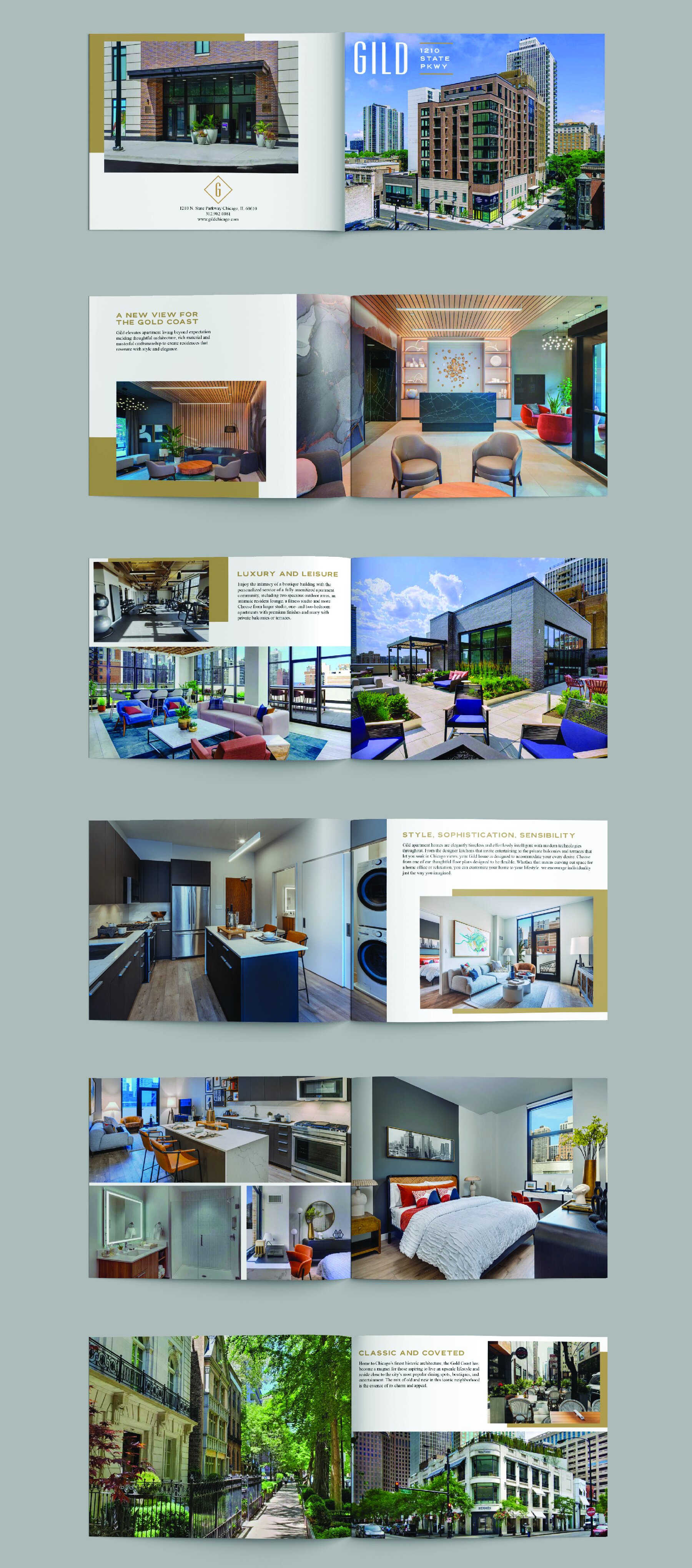The visual presentation consists of multiple colorful photographs set against a gray background, meticulously showcasing various aspects of an apartment building named Guild 1210 State Parkway. 

**Top Section:**
- The leading image captures the exterior of a towering apartment building, albeit with some illegible text beneath it. 
- Adjacent to this, on the left, is another photograph of the same building, clearly labeled "Guild 1210 State Parkway."

**Middle Section:**
- The central portion features an image of a tastefully furnished living room with dark gray walls, accompanied by the phrase "A new view for the Gold Coast," though some text beneath it is blurred and not readable. 
- To the right, a beautifully decorated room filled with potted plants and various pieces of furniture is showcased. A sleek marble reception desk adds a touch of luxury, with the caption "luxury and leisure" prominently displayed. 

**Further Down:**
- Next, a photograph of a gym is presented, followed by an impressive picture of a spacious area overlooking a vibrant city skyline, furnished with multiple couches and chairs.
- There is an image of an outdoor terrace adorned with numerous plants, tables, and chairs. The terrace offers a stunning view under a blue sky with scattered clouds, indicating a high vantage point due to the visible positioning of surrounding buildings. 
- A detailed kitchen is shown next, featuring stainless steel appliances, dark wooden cabinets, and a dark blue kitchen island with a white countertop. A stacked washer and dryer are visible on the edge of this image, accompanied by the words "style, sophistication, sensibility," though the caption beneath is too blurry to read. 

**Lower Section:**
- Following this, there is a photograph of a richly furnished living room, an elegant kitchen, a modern bathroom, and a cozy bedroom.
- A larger image of a bedroom is also included, where tall buildings are visible through the window. The bedroom contains a large bed, possibly a king or queen size, dressed in a white comforter with red and blue pillows against the headboard. 
- The bottom row features images of a sidewalk flanked by numerous buildings on one side and lush trees on the other. The caption "classic and coveted" accompanies a final image of a large white apartment building, suggesting its desirable and timeless appeal.

This comprehensive encapsulation paints a vivid picture of the luxurious living experience offered at Guild 1210 State Parkway, highlighting its various amenities, sophisticated interiors, and prime location.